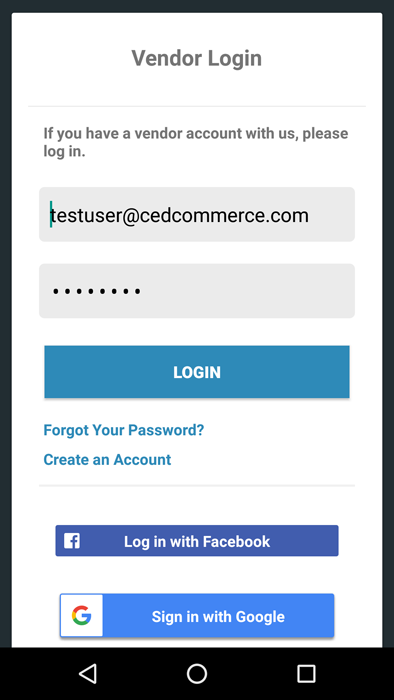The image depicts a phone screen displaying a vendor login page, characterized by a user interface with a clean white background bordered by the black edges of the phone. At the top, the text reads, "If you have a vendor account with us, please log in." 

Below this instruction, login credentials have been entered: the username "testuser@cedcommerce.com" and a password represented by a series of dots. These inputs are housed within two gray boxes. 

Beneath these fields, a prominent blue button with white text invites users to "Log In". Further options are presented in blue text: "Forgot your password?" and "Create an account", separated by a faint gray divider.

The section below offers alternative login methods. A dark blue button features a white Facebook logo and the text "Log in with Facebook". Next, a similar button—with a white left segment displaying Google's multicolored "G" logo—reads "Sign in with Google" in white letters on a blue background.

At the very bottom of the screen, navigation icons appear: an arrow pointing left on the left side and a square on the right side, likely representing a back function and a home button, respectively.